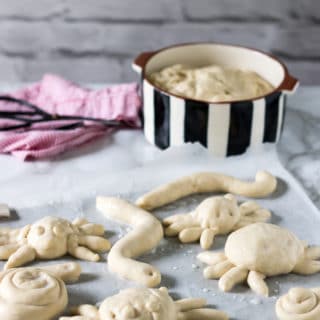A meticulously arranged kitchen counter serves as the backdrop for an engaging scene, featuring an array of dough-crafted creatures. Centered prominently is a distinctively styled ceramic pot adorned with vertical white and black stripes. To its left, a pink cotton cloth or napkin, accented with black trim or possibly draped with a black utensil, adds a splash of color to the composition. In the foreground, an assortment of whimsical dough figures captures attention. Among these creations, there are snakes elongated and curved, turtles and crabs intricately shaped, alongside some abstract forms resembling croissants with modest swirls. The overall tableau blends artistry with culinary creativity, producing a visually captivating display.